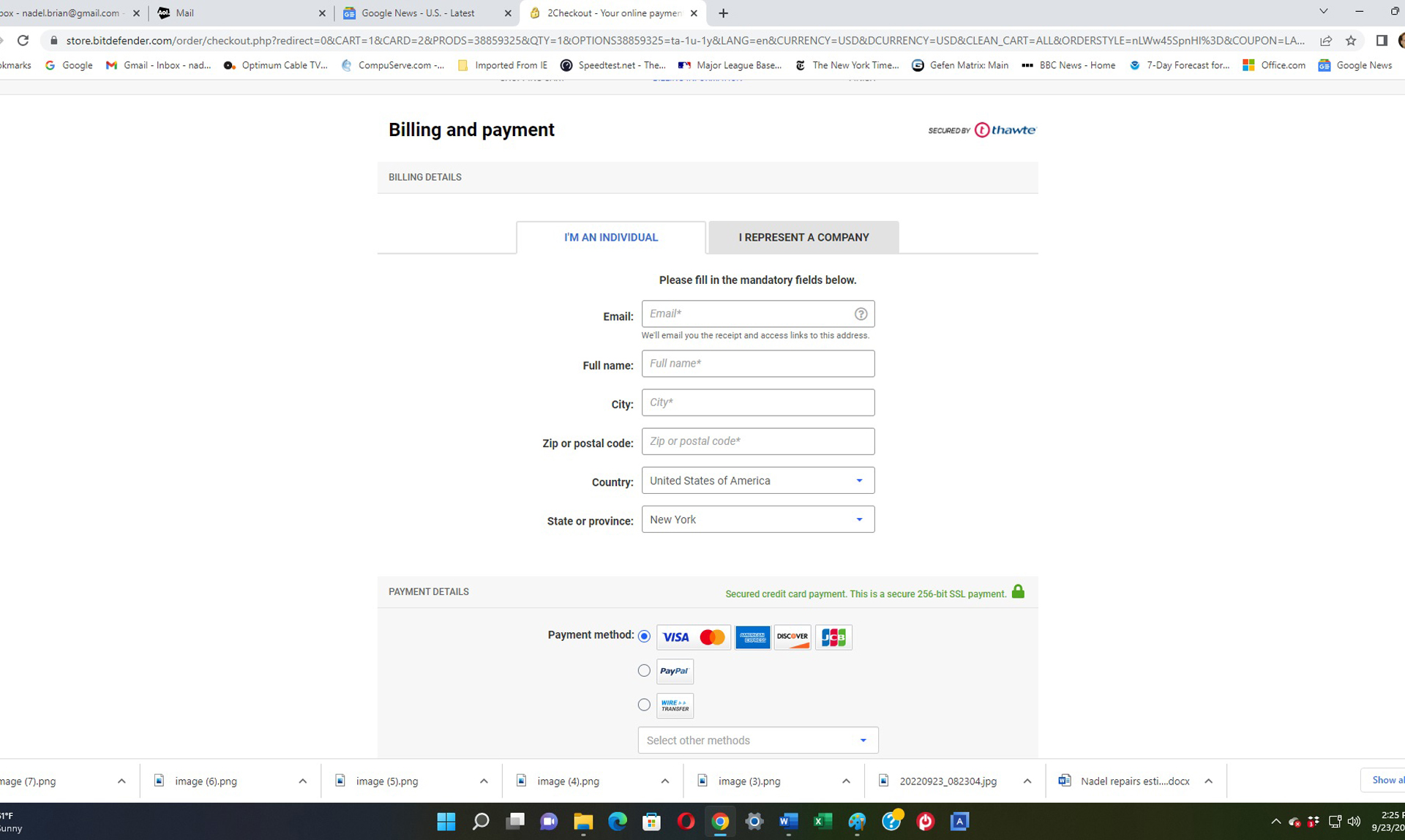This screenshot captures a browser window with four open tabs, the last one titled 'Check Out'. The browser interface includes an address bar, below which lies an extensive row of bookmarks. The currently active page is titled 'Billing and Payment,' featuring two primary tabs: 'I'm an Individual' and 'I Represent a Company.' The 'I'm an Individual' tab is selected.

Within this tab, users are prompted to complete mandatory fields such as: Email, Full Name, City, Zip/Postal Code, Country (set to 'United States of America'), and State/Province (set to 'New York'). Below these fields is a section labeled 'Payment Details.' On the same line, to the right, there’s a green box indicating a 'Secured 256-bit SSL Payment' with a padlock icon for security.

The payment method options include a first row highlighted in blue, featuring Visa, MasterCard, American Express, Discover, and JCB. Additional options are PayPal, Wire Transfer, and other methods. At the bottom of the page, there is a row of image thumbnails in JPG format with a 'Show All' button on the far right side.

The screenshot also includes the desktop toolbar, displaying numerous icons such as Chrome, Settings, Excel, PowerPoint, and a video icon, alongside a search bar and the Windows start button. To the far right of the desktop toolbar, the current time and date are visible.